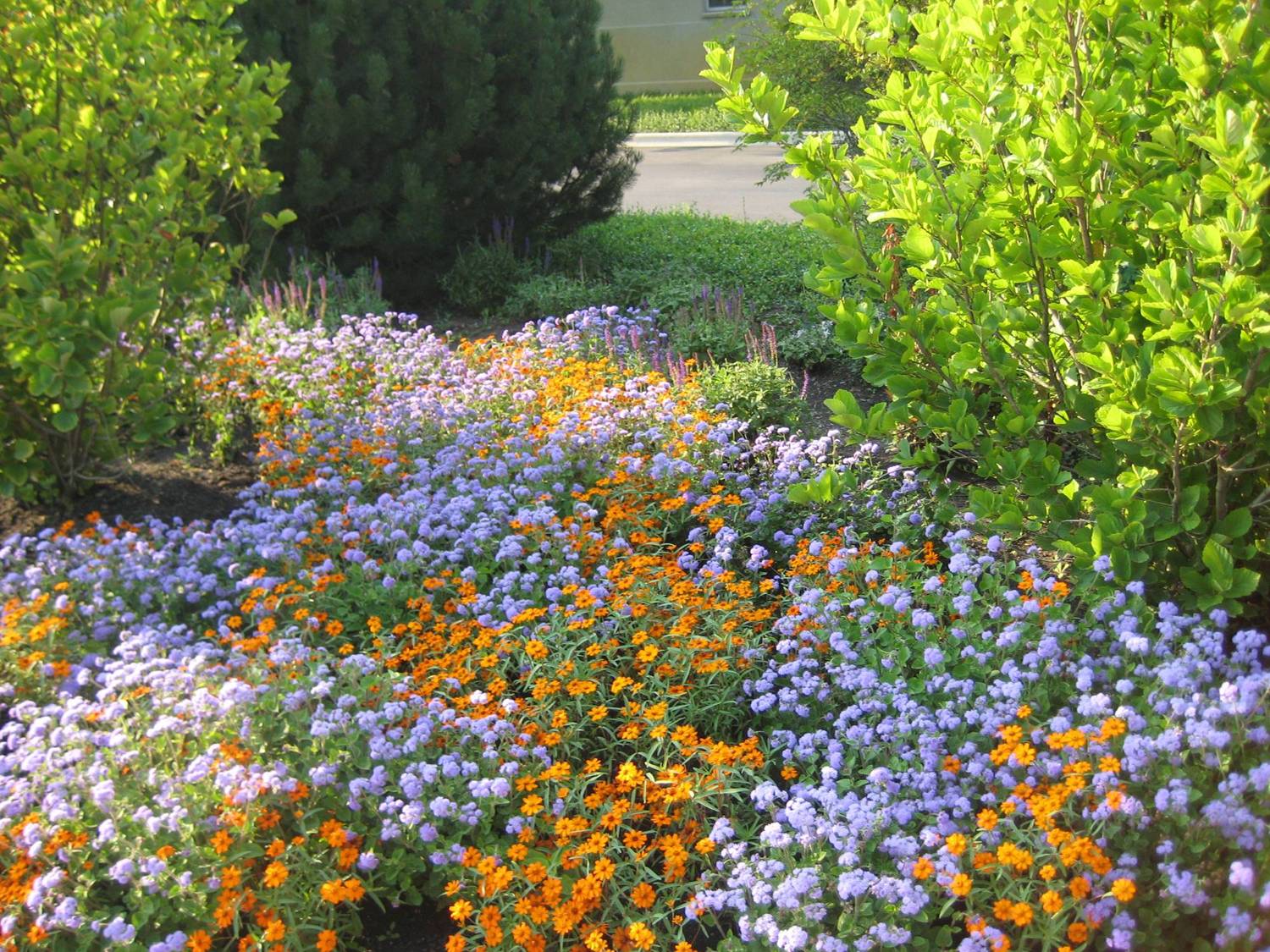This is a detailed photograph of a vibrant, landscaped garden situated in front of a house or building. In the foreground, a lush array of flowers with distinct patches of colors—purple, lavender, orange, white, and yellow—blankets the area, creating a visually appealing mix. The flowers are grouped by color, with sections of orange and purple interspersed with areas of white and small patches of yellow. Toward the right-hand side of the photo, there's a lighter green bush, while the left side features two bushes: one lighter green bush at the corner and another darker green bush in shadow toward the top left, intensifying its color. The middle of the scene is dominated by another dark green bush. The background shows a glimpse of a road with a white curb and a small grassy area beyond it. The photograph includes tall trees and additional green grass near the road, adding depth to the landscape. The dense floral coverage spreads out like a compact, colorful field, accentuating the garden's beauty and complexity.